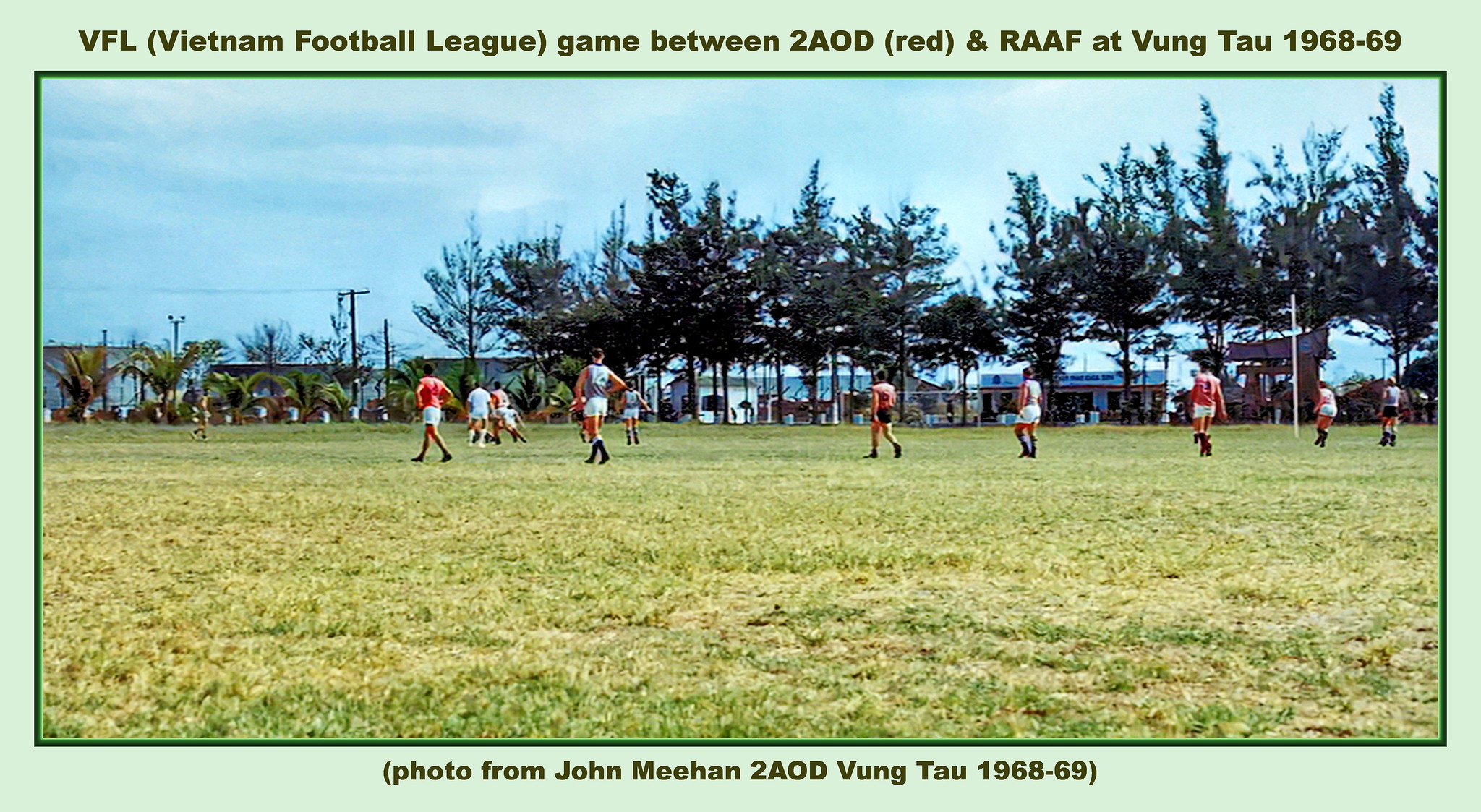This is an old, rectangular, full-color photograph, slightly faded and framed with a light gray outer border and a darker green inner border. At the top, across the blue section of the border, it reads in dark green font: "VFL, Vietnam Football League, game between 2 AOD (in red) and RAAF at Vung Tau, 1968-69." The bottom gray border includes the text: "Photo from John Meehan, 2 AOD, Vung Tau, 1968-1969." The image depicts an open grass field with patches of yellow and brown, where a soccer game is taking place. The players are mostly in red and white uniforms, with some individuals in black shorts. The field is surrounded by tall, dark green trees, and the background features a few low buildings, telephone poles, and a visible body of water beneath a blue sky. There is no visible audience.